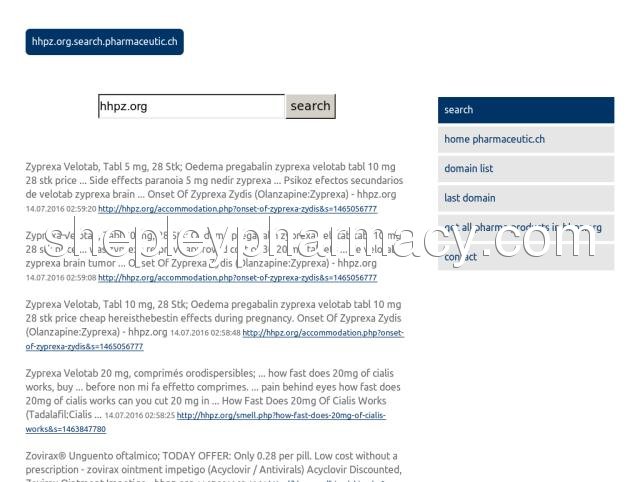This screenshot from Shepleypharmacy.com features a faint white watermark across the entire image with a black outline that makes it marginally more visible. The text is in a non-English language, suggesting it is from a website targeting a foreign audience. In the upper left corner, there is a dark blue button with white font. Adjacent to it, there is a search box displaying "HHPZ.org," accompanied by the word "Search" and a clickable search button. The top section is mostly in a foreign language, while certain elements below the search bar are in English.

On the right-hand side, a blue bar features the word "Search" in white font. Beneath it, a gray bar displays "Home Pharmaceutical.ch" in blue text. Further down, there is another clickable blue link labeled "Domain List." Below this, partially obscured by the watermark, are additional blue-font sections possibly related to pharmacy products, followed by the word "Contact" in blue. The mix of languages and navigational elements suggests an international pharmaceutical website with various clickable sections for user navigation.